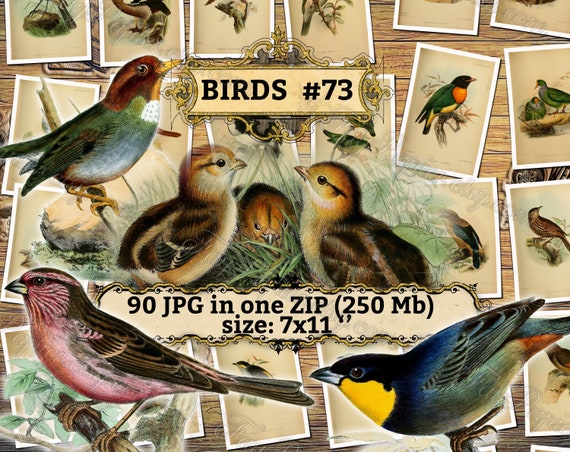This visually captivating image resembles a vintage Victorian-style advertisement, akin to nostalgic postcards. The background features an array of vintage postcards depicting various birds, laid out in a Polaroid style on a textured surface. Dominating the upper portion of the image is the inscription "Birds No. 73," adorned with intricate decorative elements that lend a labyrinthine feel.

In the foreground, artistic illustrations of birds are prominently superimposed. Centrally positioned is a bird with a brown head and a striking blue-green body. To the lower left, a pink-chested bird with a detailed face and wings is vividly portrayed. The right side showcases a bird with a yellow throat, its body primarily blue and green, and a brown tail.

Supplementing these rich visual details, the bottom of the image contains textual information: "90 JPEG in one zip, 250 MB, size 7 x 11." This suggests a collection of artistic bird images available for download, reminiscent of a curated selection from a bird-watcher's scrapbook.